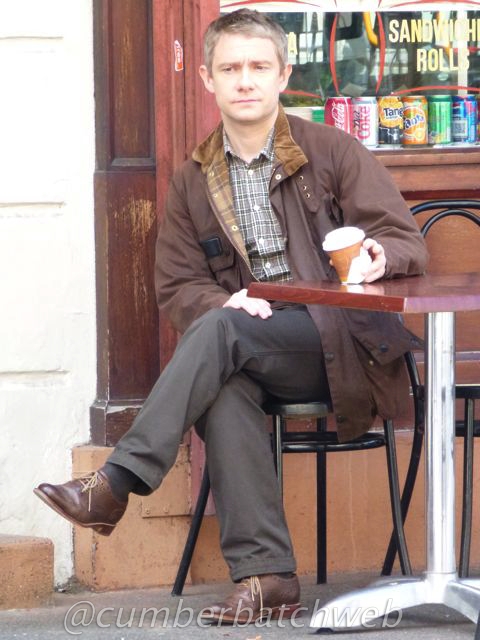In this image, a Caucasian man is seated at an outdoor table of a cafe or sandwich shop. He is wearing a brown jacket that resembles a Carhartt, a plaid button-down shirt, and khaki pants paired with brown shoes. The table he sits at is brown with a silver leg, and he sits in a black chair with his legs crossed. Holding a to-go coffee cup in his left hand, which also rests on the table, he faces slightly to the left but is mostly shown head-on. Behind him, the large storefront window displays the text "sandwich rolls," with an assortment of soft drink cans, including Coke, Diet Coke, Fanta, and Sunkist, lined up at the bottom. He appears to be observing his surroundings, possibly watching people or traffic go by, with a slightly puzzled expression on his short-haired face.